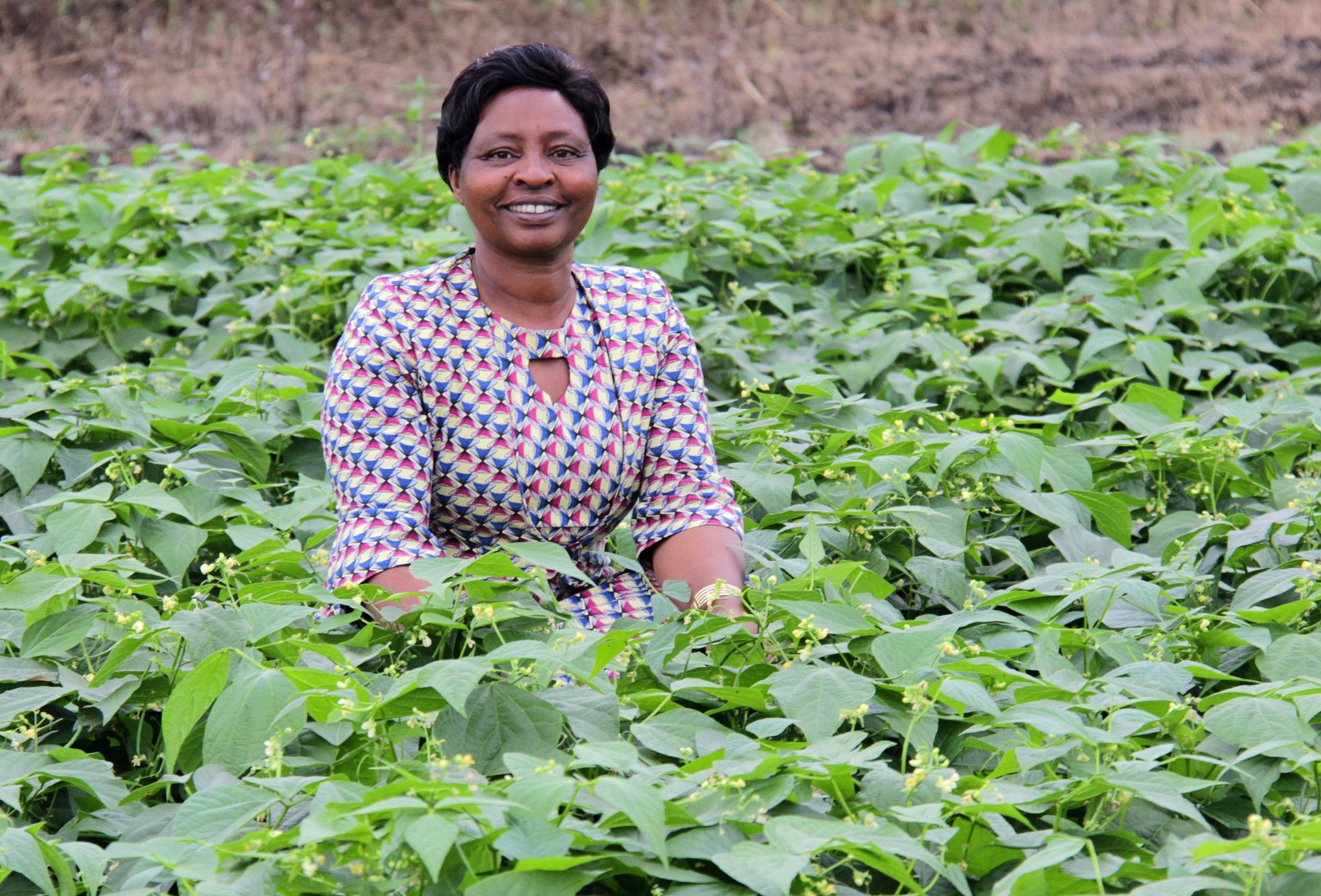In the image, a woman of South African descent with short black hair is smiling directly at the camera while squatting in a patch of lush green vegetation, which features numerous stems and leaves with budding white and yellow flowers. She is dressed in a vibrant and colorful dress adorned with a repeated pattern that starts with red at the top, transitions into a yellow center, and ends in blue, creating a striking contrast against the green backdrop. The woman is at the center of the composition, clearly the focal point, with her dress and cheerful expression drawing attention. In the background, the landscape changes dramatically; it appears untended with a mix of brown and orange hues, suggesting either dead or dormant foliage, or tilled soil, giving a slightly blurred and faded look, emphasizing the vibrant life in the foreground. The image is taken during the day, capturing the natural light that further highlights the beauty of the scene.